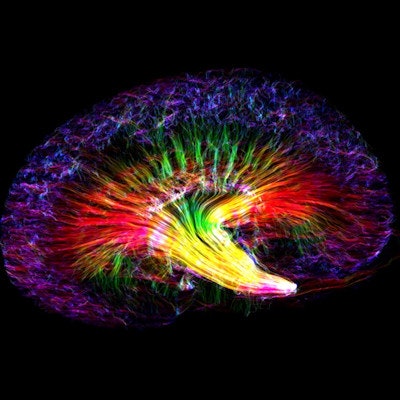The image is an abstract illustration reminiscent of the top flower of a dandelion, a blooming flower, or even the bottom side of a mushroom. At its core, there is a vivid yellow center that catches the eye with its brightness. Surrounding this center, red and green streaks create an intricate pattern, suggesting the texture and complexity of brush strokes. As the design radiates outward, it transitions into purples and blues, forming fractal-like patterns that enhance the sense of depth and movement. These colors seem to meld together in swirls that wrap around the outer edges of the artwork, creating a striking contrast against the stark black background. The overall effect is a mesmerizing blend of colors and shapes that evoke natural and organic forms in a vibrant display.